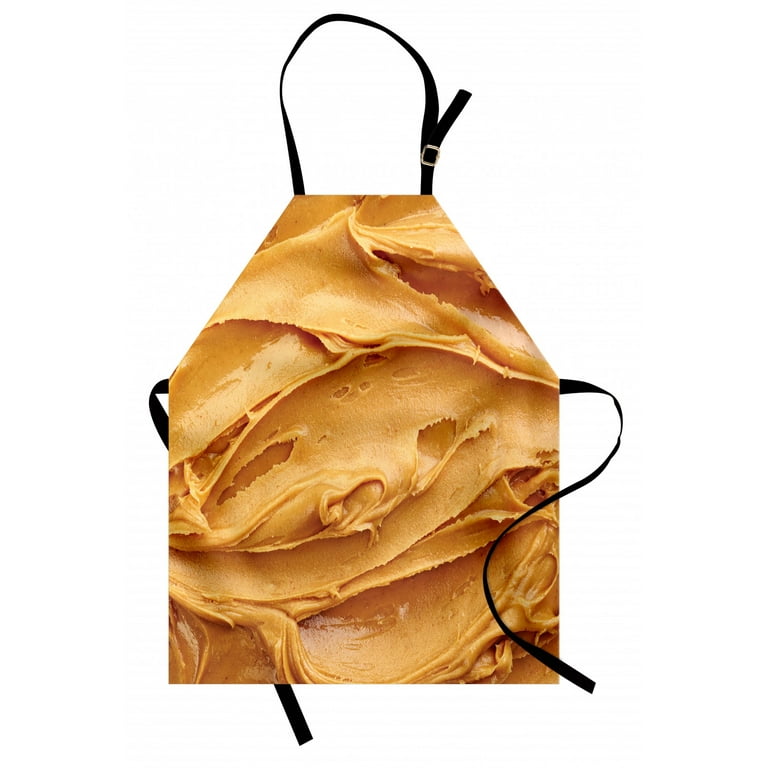The image depicts a computer-generated representation of an apron, characterized by its minimalistic and abstract design. The contours of the apron are geometrically precise, with the bottom two-thirds forming a square with three straight edges, while the top section is shaped like a slanting, flat-topped pyramid, culminating in a six-sided figure. The apron features black straps for securing around the neck and the back, with an adjustable metal component at the top for size customization. The focal point of the image is a highly detailed, close-up photograph of swirled peanut butter, giving the apron a rich, brownish-beige color with varied reflections and patterns, suggesting a half-liquid, half-solid texture. The apron is presented against a white, transparent background, emphasizing its creative and smart design suitable for kitchen use.